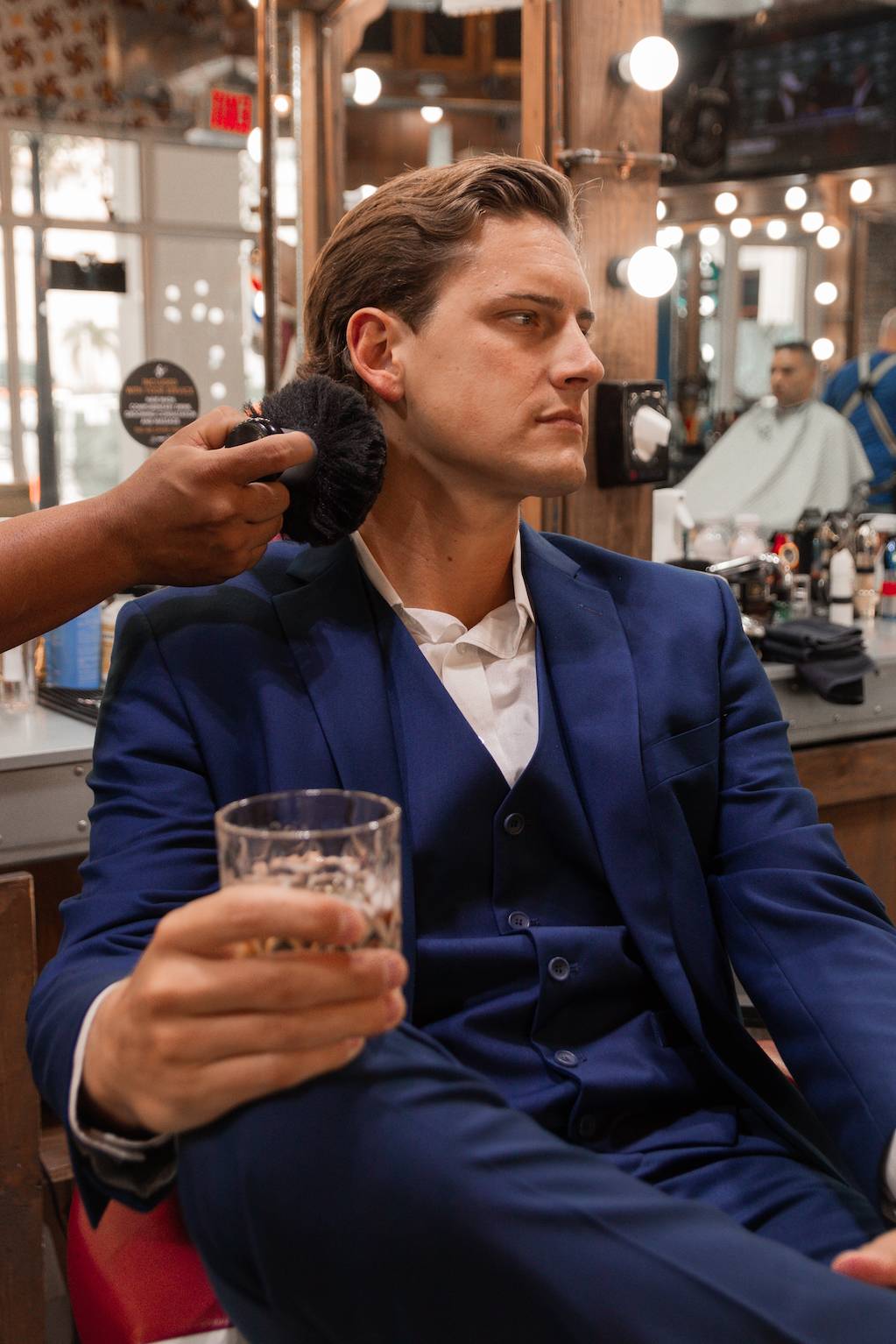In a brightly lit, classic men's barbershop, a striking color photograph captures a man in his thirties, sharply dressed in a dark blue three-piece suit with a crisp white shirt. Seated on a red stool with one leg crossed, he holds a whiskey tumbler in his right hand, exuding an air of stern confidence and a hint of arrogance. The man gazes away from the viewer, his expression serious and contemplative. A barber, possibly a person of color, is seen in the act of dusting the man's neck with a large powder brush, suggesting the recent completion of a haircut. The barbershop is bustling with an array of hairdressing accessories and mirrors reflecting various scenes, including another client draped in a traditional barbershop cape. The ambient lighting and meticulous details give the sense of a movie set, hinting that the man could be a famous actor preparing for a film or a major event.